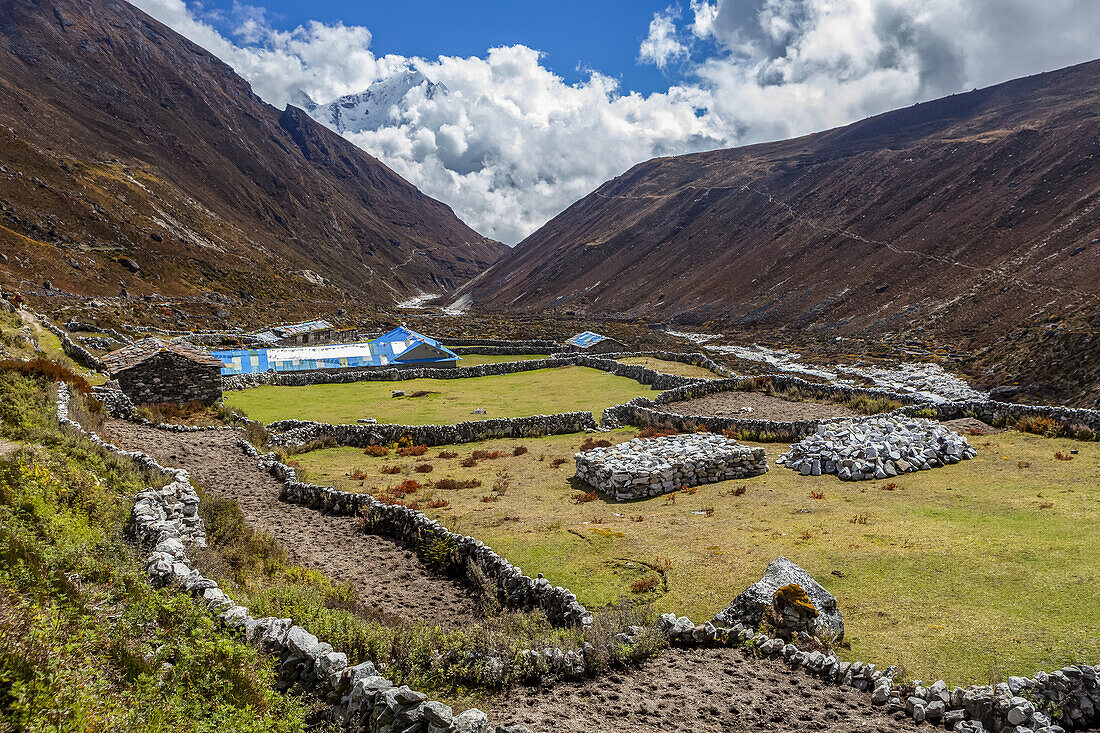This photograph captures a stunning high mountainous valley scene. On either side of the image, there are imposing, dark brown hills, smooth and rocky, sloping down towards the center to form a point, creating a natural valley. Above these hills, the sky showcases a beautiful deep blue hue, interspersed with large, billowy white clouds, and a hint of a snow-capped peak in the distant background.

The valley floor is scattered with an intricate network of low stone walls and irregular piles of gray and white stones. These stone formations create various sections within the pale yellow-green grassy expanse. Among the stone walls, a solitary sheep can be seen, adding a touch of life to the otherwise rugged landscape.

In the background, a blue-roofed industrial-type building stands out, possibly adorned with solar panels and a white sign that's not quite legible. Nearby, there is a small brown shack and a gray barn with blue writing, further accentuating the functional yet rustic appeal of the scene. The photo as a whole conveys a sense of isolation and rugged beauty, highlighting the rocky and somewhat barren nature of the valley.